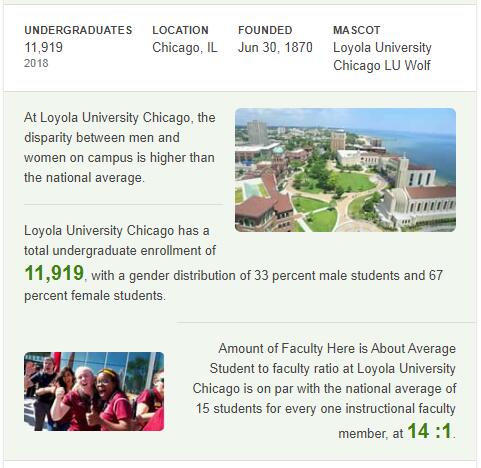The image depicts a section of a webpage featuring information about Loyola University Chicago. At the top, there's a white banner with black text reading "Undergraduates." Directly below, it specifies the number of undergraduates as "11,919 in 2018," followed by details such as the location "Chicago, Illinois," the founding date "June 30th, 1870," and the mascot "Loyola University Chicago L.W. Wolfe."

The background beneath the banner transitions into a green-gray hue. The first section states, "At Loyola University Chicago, the disparity between men and women on campus is higher than the national average." Accompanying this text is an image capturing the university campus, featuring the sky, some water, buildings, land, and grass.

Further down, additional information reveals that "Loyola University Chicago has a total undergraduate enrollment of 11,919 with a gender distribution of 33% male students and 67% female students." 

Continuing below, there's an image of a campus building with steps leading up to it, where a group of students is gathered. They are smiling and laughing. Adjacent to this image, the text outlines faculty details, stating, "The amount of faculty here is about average. The student to faculty ratio at Loyola University Chicago is on par with the national average of 15 students for every one instructional faculty member, at 14 to 1."